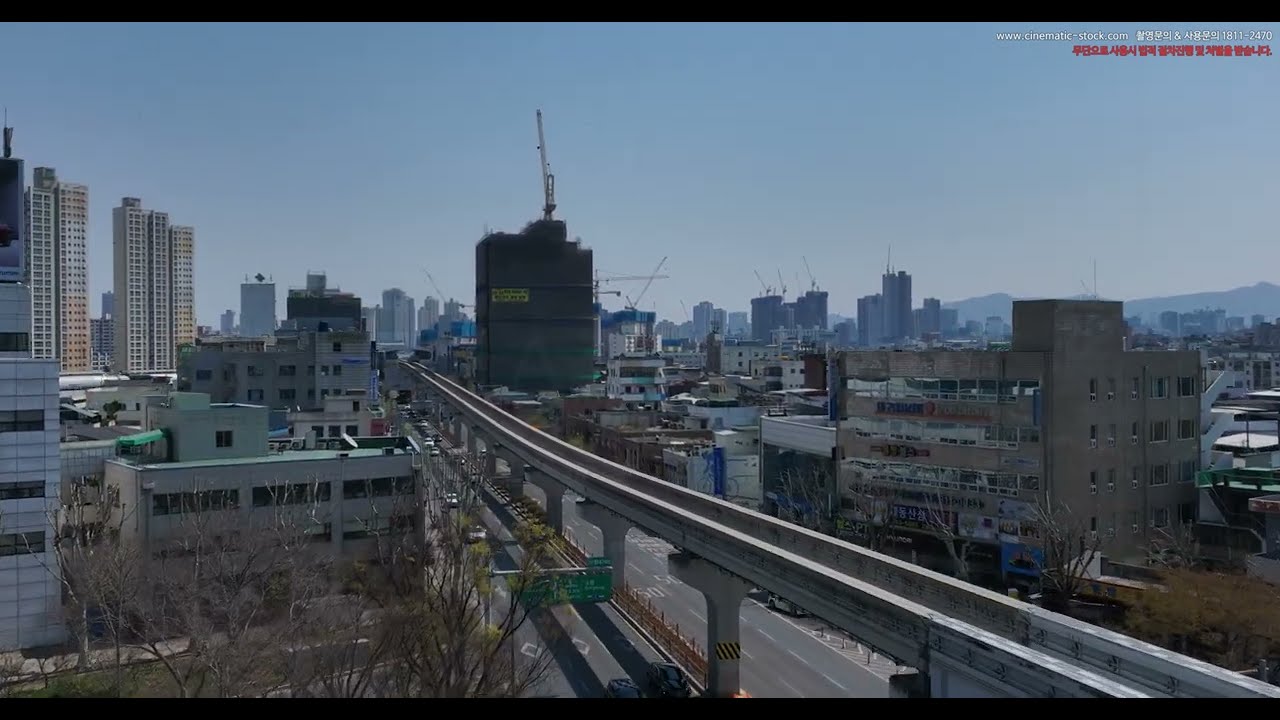The image depicts a densely populated urban cityscape during the middle of a slightly murky day. The scene features a mix of tall skyscrapers and shorter buildings primarily in tan or gray hues, interspersed with several cranes atop structures, suggesting ongoing construction. The focal point is a towering black building equipped with a crane holding metal beams, dominant amidst the shorter edifices. There are mainly leafless trees towards the left bottom center of the view, adding sparse greenery to the concrete setting.

From the bottom right corner of the image, an elevated monorail track supported by smooth, tall cement pillars snakes slightly towards the center and then upwards to the left, disappearing out of sight. This track divides the view, with various buildings creeping around it. In the distant right background, mountains are visible, adding a serene contrast to the bustling urban construction.

On the left side, more buildings rise, with a few white-walled apartment complexes that appear slightly rusty at the bottom. There's an HOV lane symbol visible on one of the streets, along with Asian lettering, hinting at the city being located possibly in China or Japan. Overall, the city scene is marked by high-rise density and a sense of continuous development.